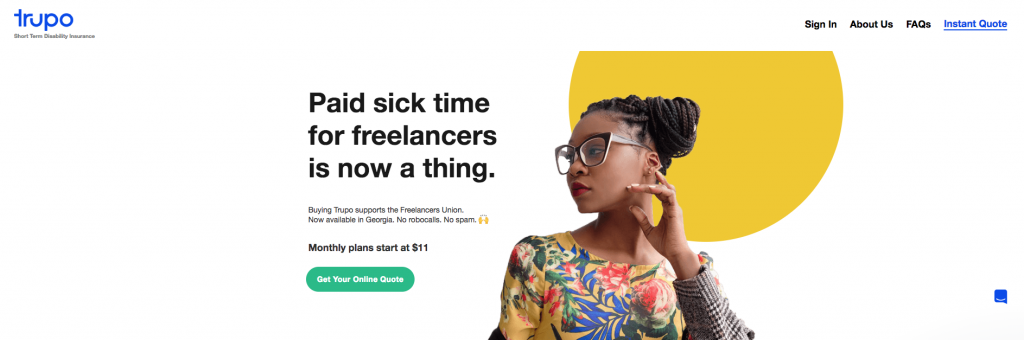At the top left of the image, there is a logo with the text "TRUPO" in dark blue, arranged in a circular, quirky font. Directly below this, in smaller black text, it reads "Short-term disability insurance," although the font size makes it somewhat hard to read. 

The center of the image features a black woman with dreads styled into a side bun. She is wearing retro glasses and a floral dress, with her left hand thoughtfully placed near her face. Her gaze is directed to the side. To the left of her, bold black lettering reads, "Paid sick time for freelancers is now a thing."

Below this statement, smaller black text informs the reader: "Buying TRUPO supports the Freelancers Union. Now available in Georgia. No robocalls, no spam," accompanied by the praising hands emoji. Another bold message beneath this declares, "Monthly plans start at $11."

A green oval icon at the bottom of the image bears the text "Get your online quote" in white letters. There is a large mustard-yellow circle partially obscured behind the woman's hair and head, adding a vibrant background element.

At the top right corner, a black-bold menu provides options labeled "Sign In," "About Us," and "FAQs." Additionally, to the far right, a blue underlined text reads "Instant Quote." In the bottom right corner, there is a message box icon indicating that users can start a conversation with a representative.